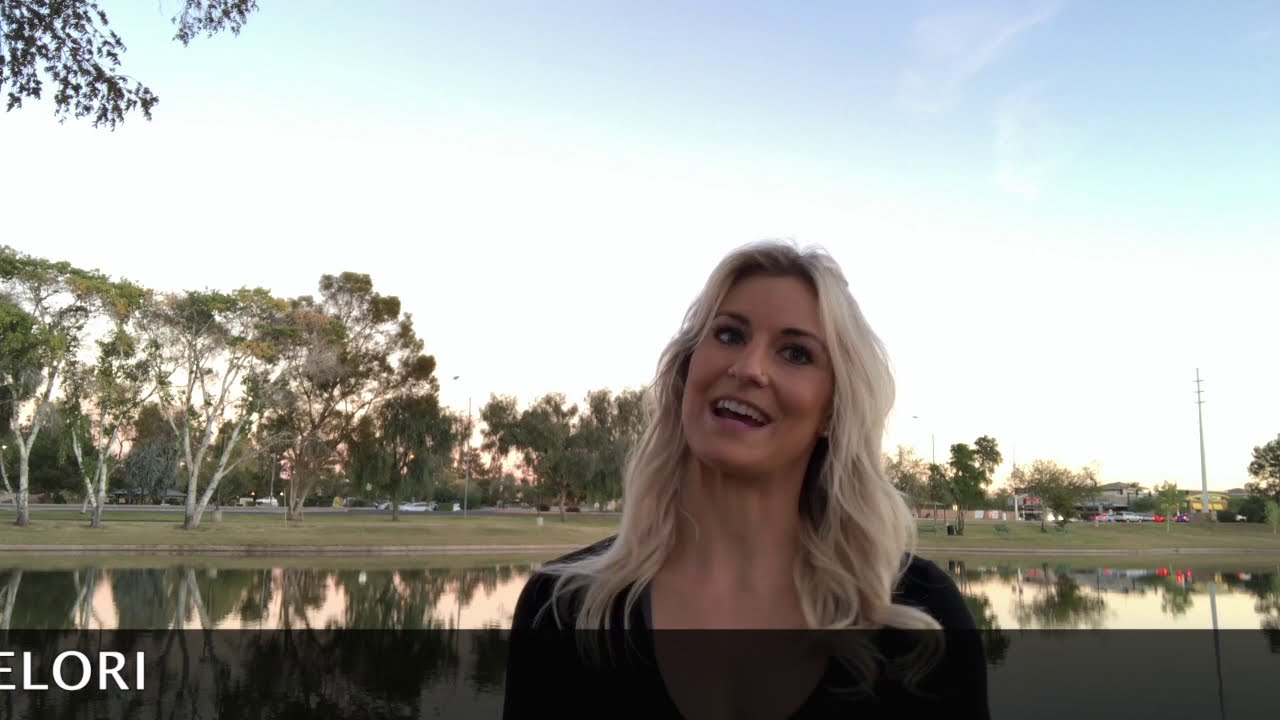In this photograph, a young Caucasian woman in her early 30s, with long, wavy, light blonde hair that falls just past her shoulders, stands in front of a serene pond. She is wearing a black scoop-neck top and is seen from the shoulders up, with her head tilted slightly back and to the right, as if mid-sentence or smiling while speaking. Notably, she has a stud on her nostril. Behind her, the still pond mirrors a lush strip of green manicured grass and a variety of large trees, some with white trunks. Farther in the background, a row of small buildings and what might be commercial businesses line the horizon. A paved walkway can be seen running along the greenbelt. To the right, a possible radio or power tower stands tall against a hazy pale blue sky with a few wispy clouds, suggesting it might be late afternoon. Adding a final touch to the image, a black band with white text reading "E-L-O-R-I" runs across the bottom, indicating this might be a snapshot from a video, perhaps of a realtor providing a tour of this suburban setting.